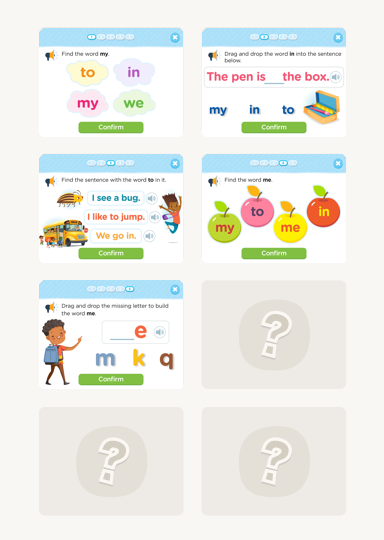The image showcases a children's educational website featuring simple learning games. The page has a light gray background and displays eight modules arranged in four rows and two columns. Currently, five of the modules are filled in, while the last three feature large question marks, indicating they may be future additions. Each filled module represents a different type of word game designed to enhance basic literacy skills for preschool children. 

For instance, one game challenges children to find the word "my" among several cloud-shaped words, requiring them to click on the correct one. Upon selecting a game, a big green "confirm" button appears, allowing the child to start playing. Another game involves filling in the blank, while a more complex one tasks players with identifying sentences containing the word "to." 

One of the modules encourages finding multiple instances of the word "me," and the last filled module is a drag-and-drop activity where children must place missing letters to complete the word "me." Each game is designed to be interactive and fun, providing an engaging way for young children to build their vocabulary and reading skills.